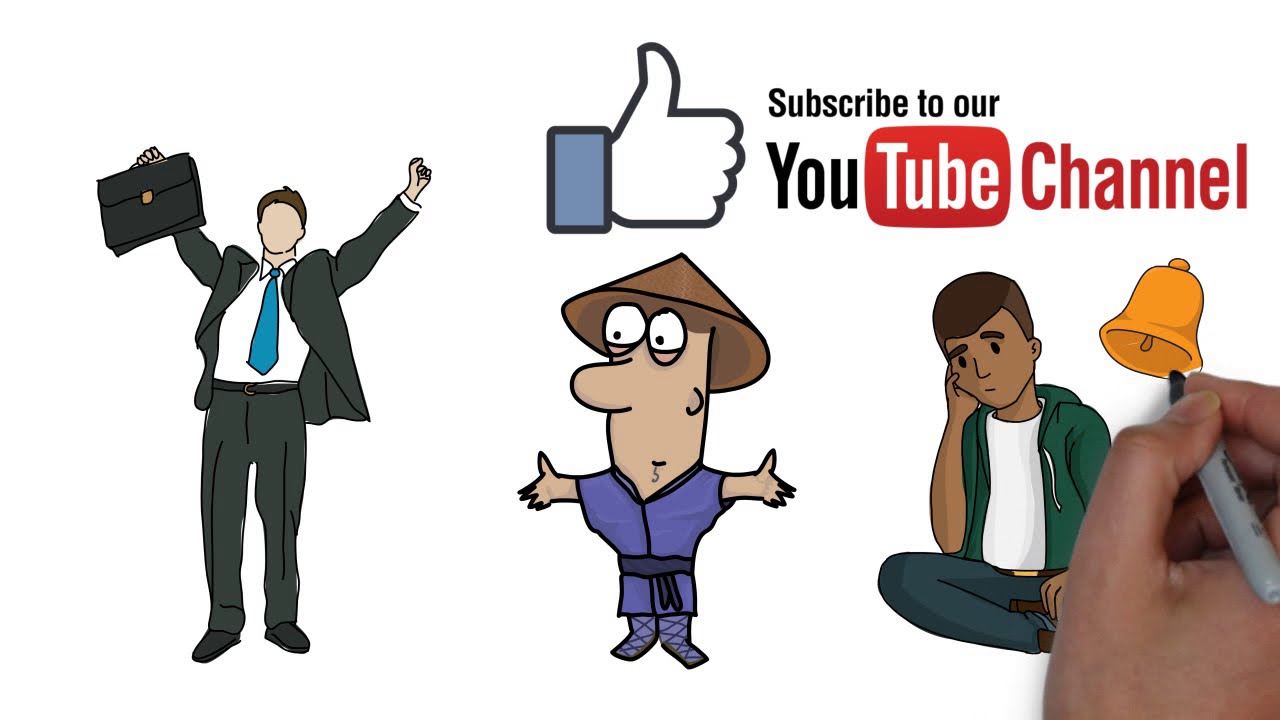The image is a vibrant collage of animated drawings and some real-life elements, featuring several distinct objects and characters. On the left side stands a caricature of a male figure dressed in a white shirt, blue tie, unbuttoned suit jacket, black belt, pants, and shoes. His arms are raised, and he's holding a briefcase, giving an impression of excitement or celebration. The central focus includes a blue thumbs-up emoji with text above it that reads, "Subscribe to our YouTube channel." Below the thumbs-up is a male caricature in a purple karate outfit with a black belt and an Asian-style hat. To the right is a male figure in a green sweater and navy blue pants, sitting in a yoga position, resting his head in one hand, appearing contemplative or upset. The final element on the right side of the image is a hand, partially photographed, holding a Sharpie marker and drawing a gold bell notification icon. The overall scene combines both digital graphics and a real photo element, bringing together various themes of enthusiasm, encouragement, and deep thought.